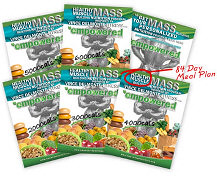This image features a small graphic on a white or transparent background, showcasing six magazine covers arranged in two rows of three. Each row features a central magazine, flanked by two others on either side, creating a symmetrical layout. The covers prominently display images of hamburgers and some text at the top, though the exact wording is unclear. Additionally, one of the magazines includes a notable circular element with an arrow pointing to it, accompanied by the text "84 Day Meal Plan." The overall appearance suggests that this graphic is a web-based visual, possibly related to a meal planning or culinary publication.